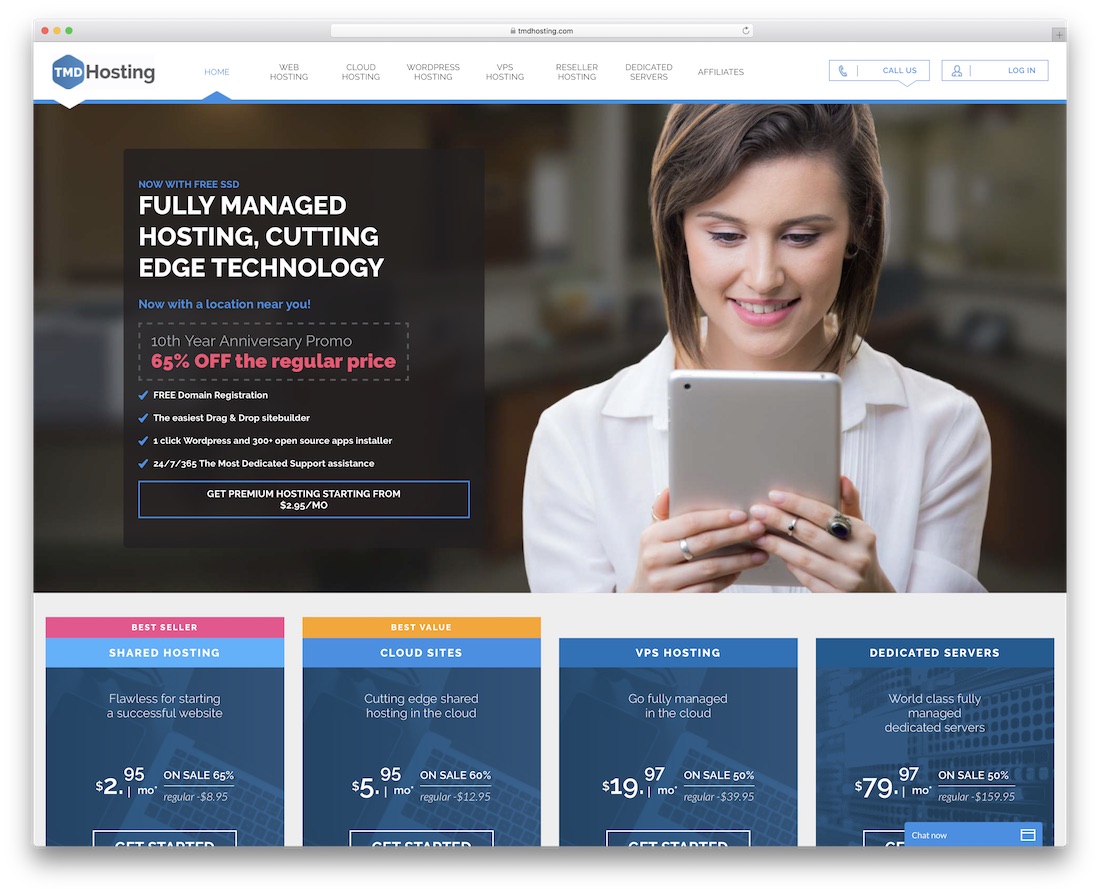This image is a detailed screenshot taken from a computer, likely a laptop or desktop, of a web browser displaying the TMD Hosting homepage. The browser's interface is visible at the top, starting with a long, thin, gray address bar featuring the URL, "tmdhosting.com". 

In the upper left corner of the browser window, familiar MacOS interface elements are visible: the red, yellow, and green circles used to close, minimize, and resize the window, respectively. Adjacent to these circles is a small, white rectangular logo of TMD Hosting, showcasing white letters on a blue pentagon background, followed by the word "Hosting" in black.

Below the address bar is the website's main navigation menu styled with a blue highlight to indicate the active selection on the "Home" tab. Other menu items include Web Hosting, Cloud Hosting, WordPress Hosting, VPS Hosting, Reseller Hosting, Dedicated Servers, and Affiliates. On the right side of this menu bar, there are icons for phone contact and user login options.

The main content area of the site features a prominently blurred background image hinting at a domestic kitchen setting, behind which a woman holds a large tablet. On the left side of this section, in a black box with white text, the site advertises "Fully Managed Hosting, Cutting Edge Technology," with a promotional message about their 10th anniversary offering 65% off the regular price.

Below this promotional banner, the site presents four blue rectangles, each highlighting different hosting plans. They include:

1. **Bestseller Shared Hosting** - with detailed information and pricing
2. **Best Value Cloud Sites** - emphasized with descriptive details and cost
3. **VPS Hosting** prices and specifications
4. **Dedicated Server** prices and features

This detailed screenshot gives a comprehensive look at TMD Hosting's website, showcasing their product offerings and promotional deals.